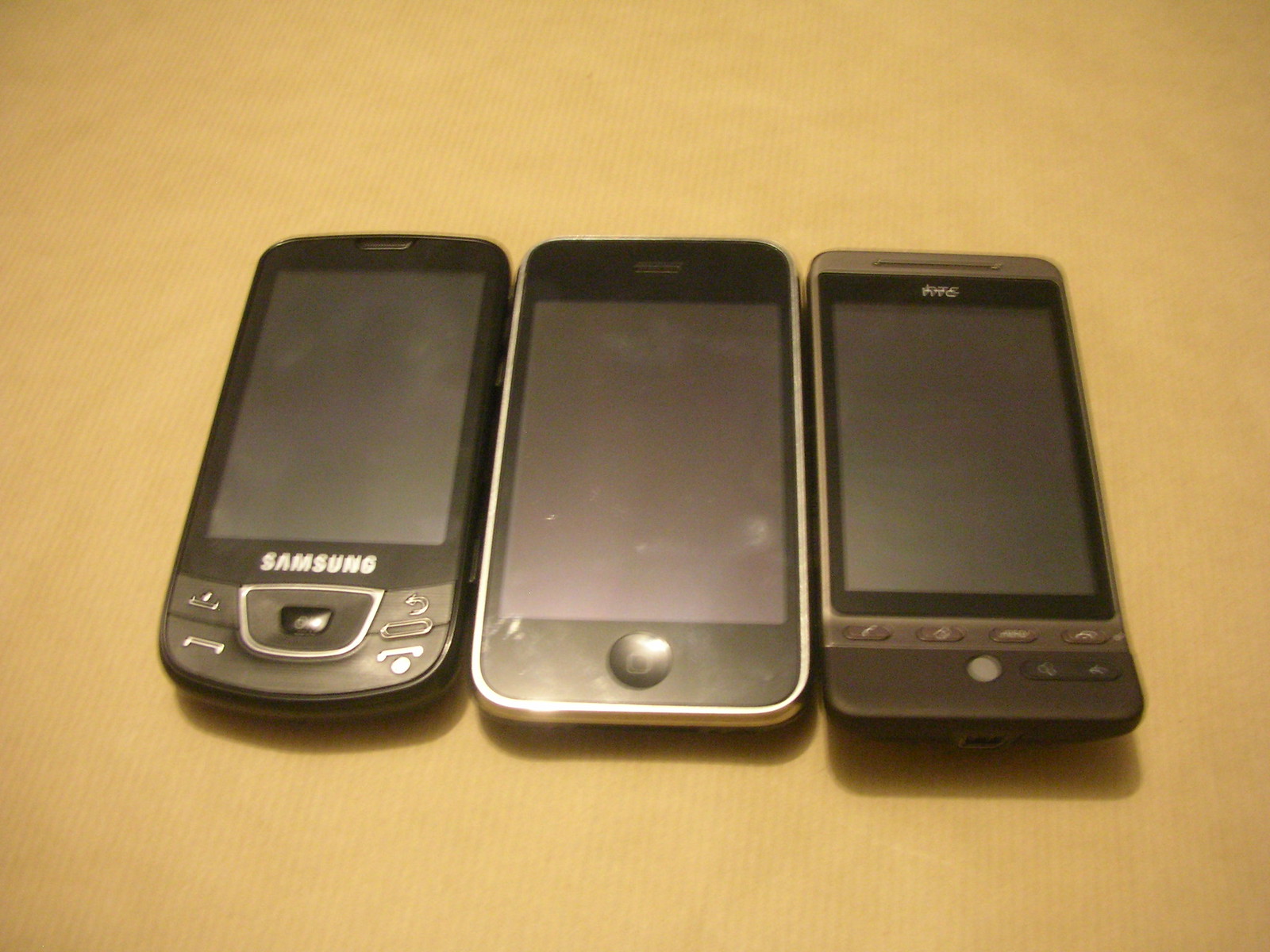The photograph showcases three old, vintage cell phones laid side by side on a bright bronze, brownish table. The one on the left is a black Samsung phone, notable for its physical keypad and central joystick, indicative of a model predating modern smartphones. The middle phone is the largest among the trio and features a minimalist design with no visible brand name, a single central button below the screen, and no additional buttons. The cell phone on the right, which is slightly smaller, leans towards a brownish hue with a brand name that is too blurry to identify. It features a larger screen with four small buttons below it, a central round button, and extra buttons to the right of the main one. All phones are switched off, as indicated by their blank screens. The overall image has light focusing on the phones, accentuating their vintage design against the beige orangy-beige textured table background.